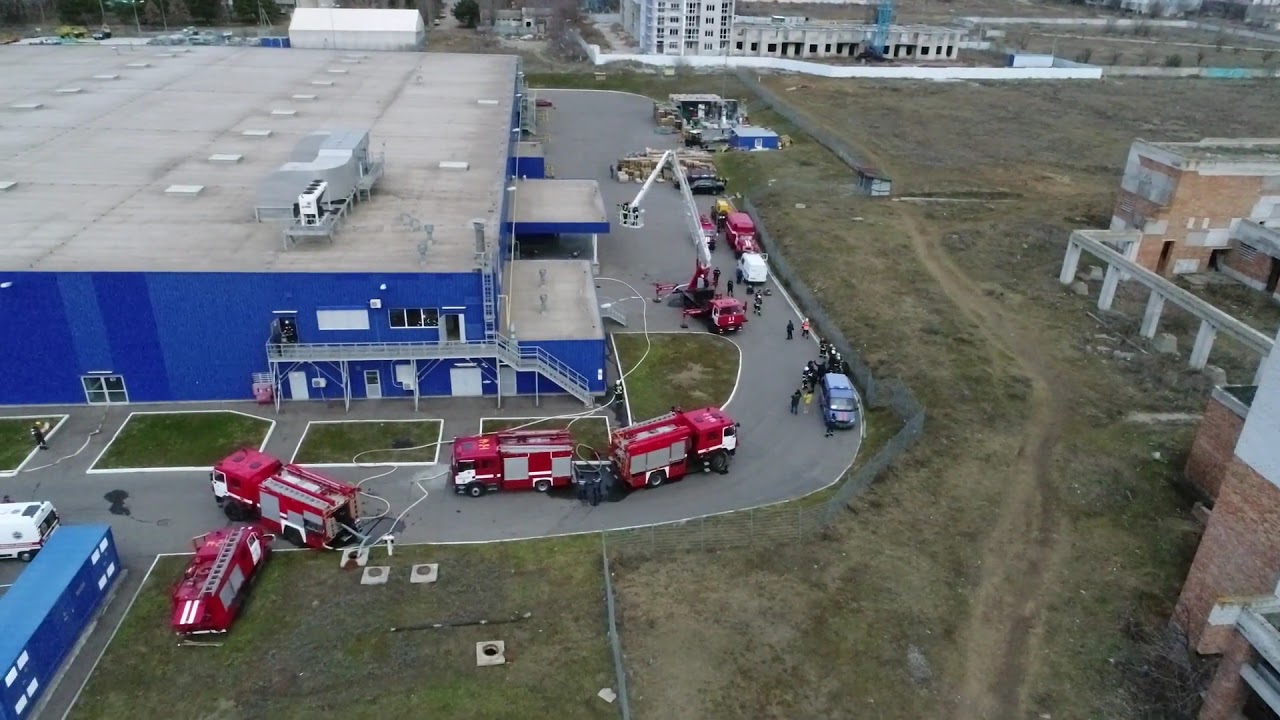The daytime aerial photograph captures a sprawling industrial area, focusing on a substantial blue building with a flat, gray roof hosting numerous air conditioning units. The structure resembles a typical large-scale supermarket. In front of the building, there is a cluttered landscape marked by a mixture of dirt and sparse grassy patches. 

Several red and gray fire trucks are stationed prominently in the driveway, their hoses out and directed towards the blue building. One notable truck features a long white boom extended into the air, carrying personnel up to the building's second story. Scattered emergency personnel and onlookers are visible around the site. To the right of the building, there is a brown brick structure supported by gray cement columns, while the upper portion of the image reveals adjacent two- and three-story gray cement buildings that enclose the area, their walls uneven and jagged.